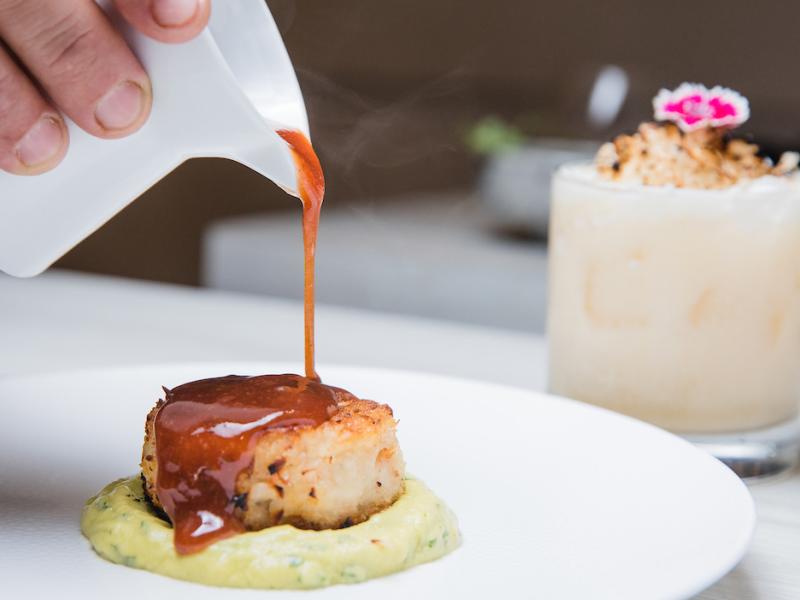In the image, a hand is seen pouring a thick, honey-colored syrup from a white cup, tilted forward, onto a small dessert below. The cup is held by two fingers visible in the top left corner. The dessert receiving the syrup is a thick, biscuit-like patty with a brown top and white sides. This patty sits on a greenish-yellow paste on a large white plate. The background is blurred, but hints of a muted brown color can be seen, with possibly a table and bowl. Off to the right, there is a white cake adorned with brown crumbles and a decorative white and red flower. The entire setting conveys a close-up, detailed view of a gourmet presentation.